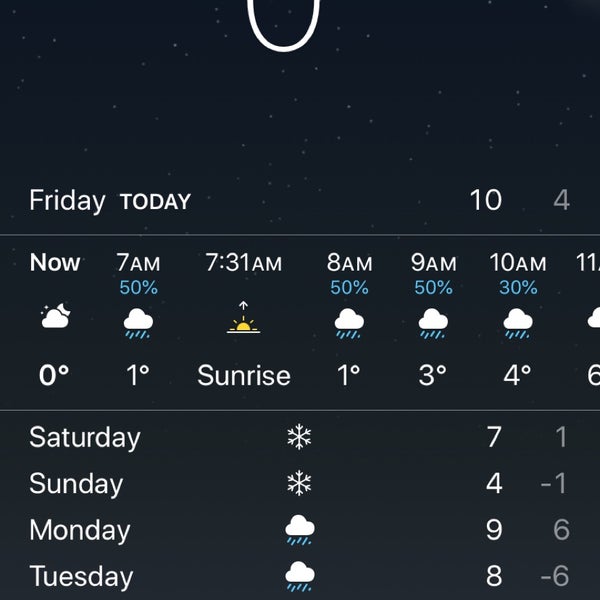**Detailed Descriptive Caption:**

The image is a screenshot capturing a portion of a webpage or a section of a cell phone screen. The screenshot is square-shaped, presenting a clipped section of a webpage more than anything else. At the very top center of the image, there is the bottom half of a large white 'O'. All the text, numbers, and icons in the image are displayed in white, creating a clear and clean interface.

On the center-left side of the screenshot, the word "Friday" is displayed, and to its immediate right, the word "Today" is in bold. On the far right of these headers, the number "10" is boldly presented, with a lighter-colored "4" adjacent to the right.

Immediately below this top section, a light gray horizontal line extends across the screen, serving as a divider. Below this line, a series of time stamps are displayed from left to right: "Now," "7 a.m.," "7:31 a.m.," "8 a.m.," "9 a.m.," "10 a.m.," and "11 a.m." Underneath each of these time indicators, weather icons are aligned. The icons from left to right are: a cloud, a cloud with blue rain lines, the sunrise, a cloud with rain lines, a cloud with rain lines, a cloud with rain lines, and finally a cloud.

Accompanying the weather icons, a row of temperatures is listed from left to right: "0°," "1°," "Sunrise," "1°," "3°," "4°," and "6°."

Below another gray divider line, five-day weather forecasts are provided on the left-hand side. Starting with Saturday, centered text indicates "Snow" with a high of "7°" and a low of "1°." For Sunday, it shows "Snow" with a high of "4°" and a low of "-1°." Moving on to Monday, a cloud with blue rain lines symbolizes rainy weather, paired with a high of "9°" and a low of "6°." The final entry is for Tuesday, which features a white cloud with blue rain lines, indicating rainy weather, with a high of "8°" and a low of "-6°."